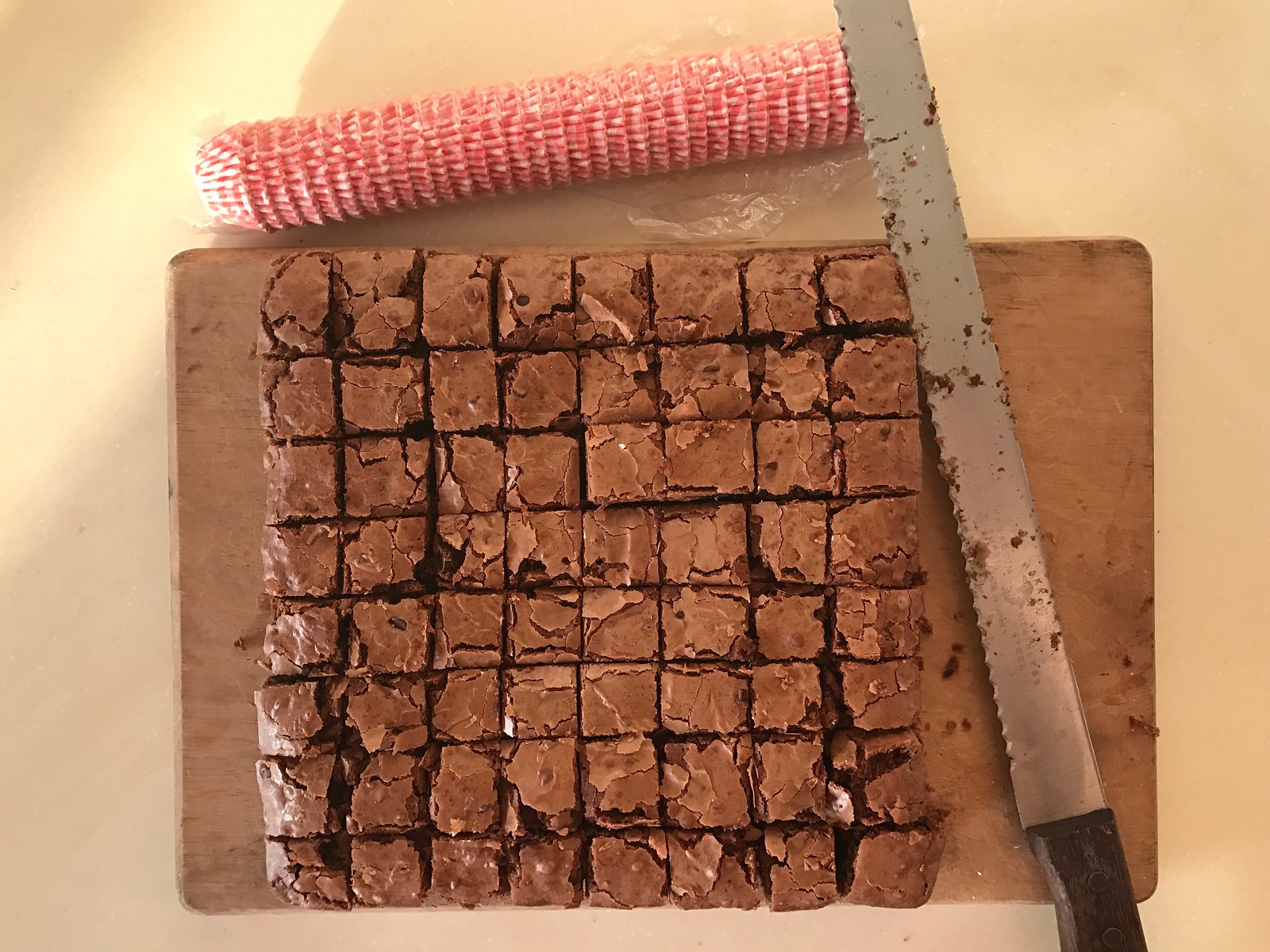In this detailed close-up photograph, we see a light brown, wood-grain cutting board resting on a tan countertop. Centered on the cutting board are 64 chocolate brownies, meticulously cut into small, even squares measuring approximately an inch to an inch and a quarter. The brownies have a rich, chocolate brown color with a slightly flaky top and dark brown specks, giving them a delectable appearance. Positioned on the right side of the brownies is a long serrated knife with a silver blade and a black handle. The knife has visible chocolate crumbs on the blade from cutting the brownies. Resting underneath the tip of the knife is a cylindrical piece of pink yarn with grooves encircling it. The arrangement of objects and the detailed textures make this a visually intriguing composition.